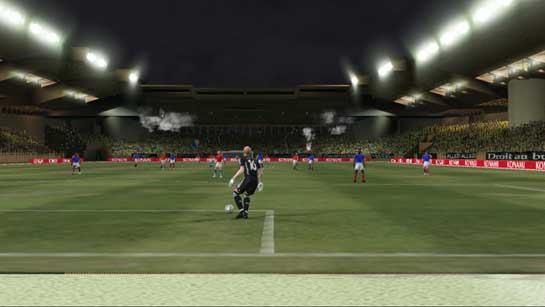The image depicts a detailed and highly realistic scene of a soccer game, potentially from a computer-generated environment or video game like FIFA. Taken from just behind and slightly to the right of the goalie’s perspective, the view centers on a black-jerseyed goalie who is positioned near the goal area, facing away from the camera. The soccer ball is resting near the white line, poised for a goal kick. In the background, a mix of players in blue and red jerseys are scattered across the lush green field. The crowded stands are visible in the upper half of the image, filled with animated fans and bathed in the glow of stadium lights against a nighttime sky. Red advertisement banners line the sides of the stands, adding color and vibrancy to the scene. The absence of the goalpost suggests it might be intentionally omitted to avoid obstructing the view, enhancing the immersive experience typical of a video game.